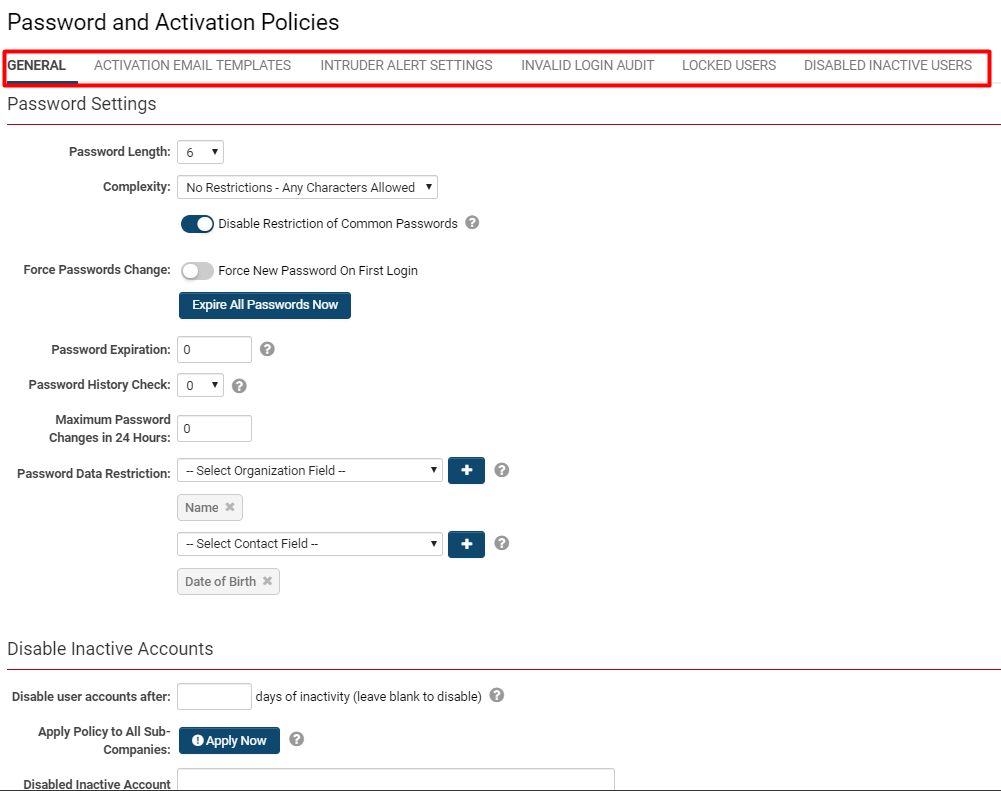**Screenshot of the Password and Activation Policies Webpage**

At the top of this webpage, we see the title "Password and Activation Policies". A prominent red rectangle encases the entire set of options at the top. Below the title, "General" is underlined and followed by several other sections in gray, including "Activation Email Templates", "Intruder Alert Settings", "Invalid Login Audit", "Locked Users", and "Disabled Inactive Users".

Highlighted by a red line that spans across the page, "Password Settings" begins with various configurations:

- **Password Length**: Minimum of 6 characters.
- **Complexity**: No restrictions; any characters are allowed.
- **Disabled Restriction**: Common passwords are permitted.
- **Force Password Changes**:
  - New passwords required upon first login.
  - A button labeled "Expire All Passwords Now" is available for immediate action.

- **Password Expiration**: Set to 0 (no expiry).
- **Password History Check**: Set to 0 (no history check).
- **Maximum Password Changes in 24 hours**: Set to 0.

Next, the **Contact Menu** and various selection fields are displayed, featuring options to add additional contact fields through a blue plus button. Specific fields include:
- "Name"
- "Date of Birth" (which can be removed if necessary).

Finally, there's a section for managing **Disabled Inactive Accounts**:
- "Disable user accounts after X days of inactivity" where X can be specified.
- Options to "Apply Policy to All Subcompanies" and an "Apply Now" button.

In conclusion, this page serves as a comprehensive security settings interface for managing login policies.